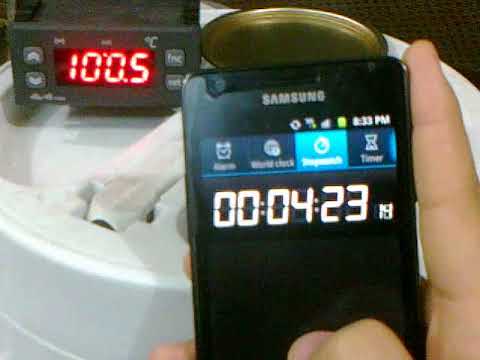The image captures a scene where a person is holding a black Samsung phone in the foreground, displaying the stopwatch feature with a time of 00:04:23 and 49 milliseconds. The phone screen shows four options at the top: Alarm, World Clock, Stopwatch, and Timer. In the upper left corner of the image, a gray device is visible. It has buttons labeled "up," "down," "FNE," and "set" on its front panel, and its display shows a glowing red reading of 100.6, likely representing degrees Celsius. Behind this device, a cooler or drink storage device can be seen, adding context to the setting of temperature and time monitoring.